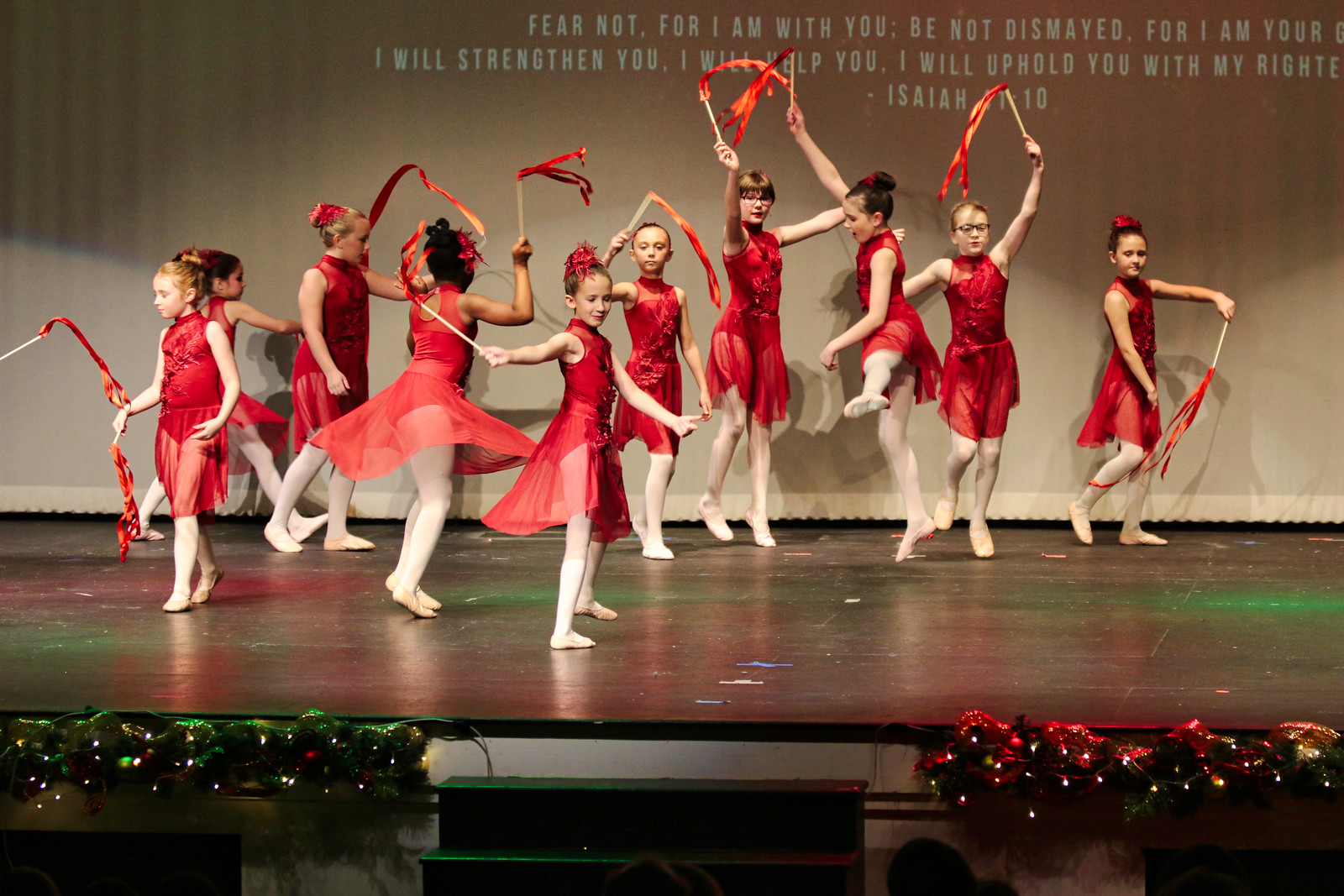The image depicts a color photograph of a performance by approximately a dozen young girls of varying heights and ages on a black wooden stage. The girls are dressed in red high-neck tank top leotards with red flowy skirts, white tights, and white ballet-type shoes. Each girl holds a white stick with a red ribbon at the end, and they are all captured in different dance positions—some with arms extended, some twirling their ribbons, and others lifting their legs.

The stage floor is illuminated by green lights along the bottom and the stage edge, with red lights shining from the right side. Small Christmas lights are visible in front of the stage, with poinsettias and evergreens adorned with lights flanking a set of steps in the middle. A beige wall forms the backdrop, adorned with a partially visible Bible verse from Isaiah: "Fear not, for I am with you; be not dismayed, for I am your God. I will strengthen you, I will help you, I will uphold you with my righteous right hand."